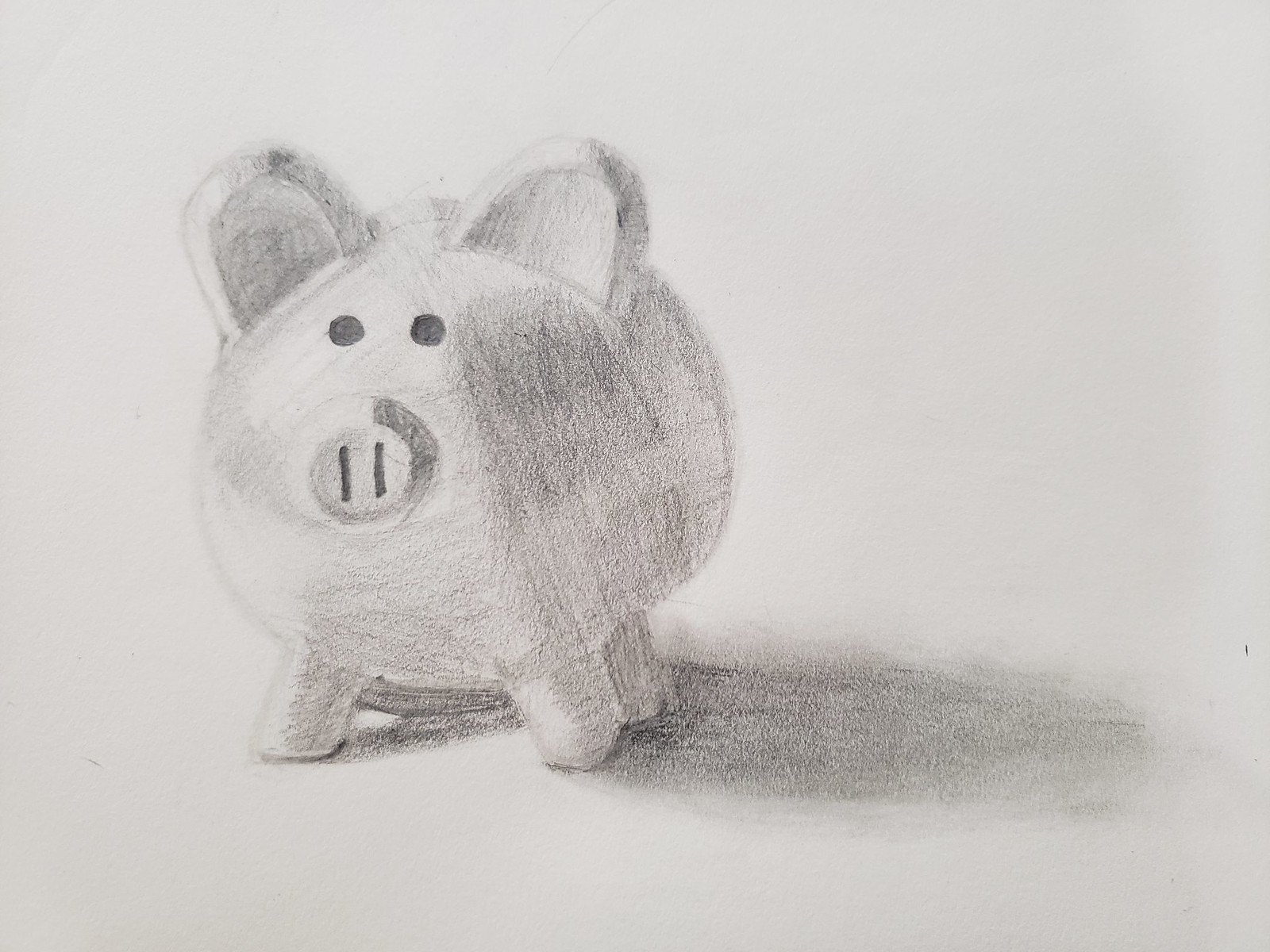The image is a highly detailed pencil sketch of a porcelain piggy bank, rendered entirely in shades of black and gray. Positioned centrally on the left third of the drawing, the piggy bank is oriented to face the viewer, showcasing its round, almost three-dimensional form with intricate shading. The pig has large, simple ears shaped like upside-down U’s, and a notable plateau-like nose with two black vertical slits that serve as nostrils, likely functioning as the coin slot. The pig’s stubby, rounded legs are visible beneath its body, though only three legs—the front two and the back left—are fully discernible due to the pig’s slight leftward tilt. It casts a shadow that extends towards the right side of the image, filling the middle right portion with a gradient of pencil shading. The background remains a plain, light gray, providing stark contrast to the darkly shaded piggy bank, and there are no other distinguishing marks or colors present in this minimalistic yet detailed representation.